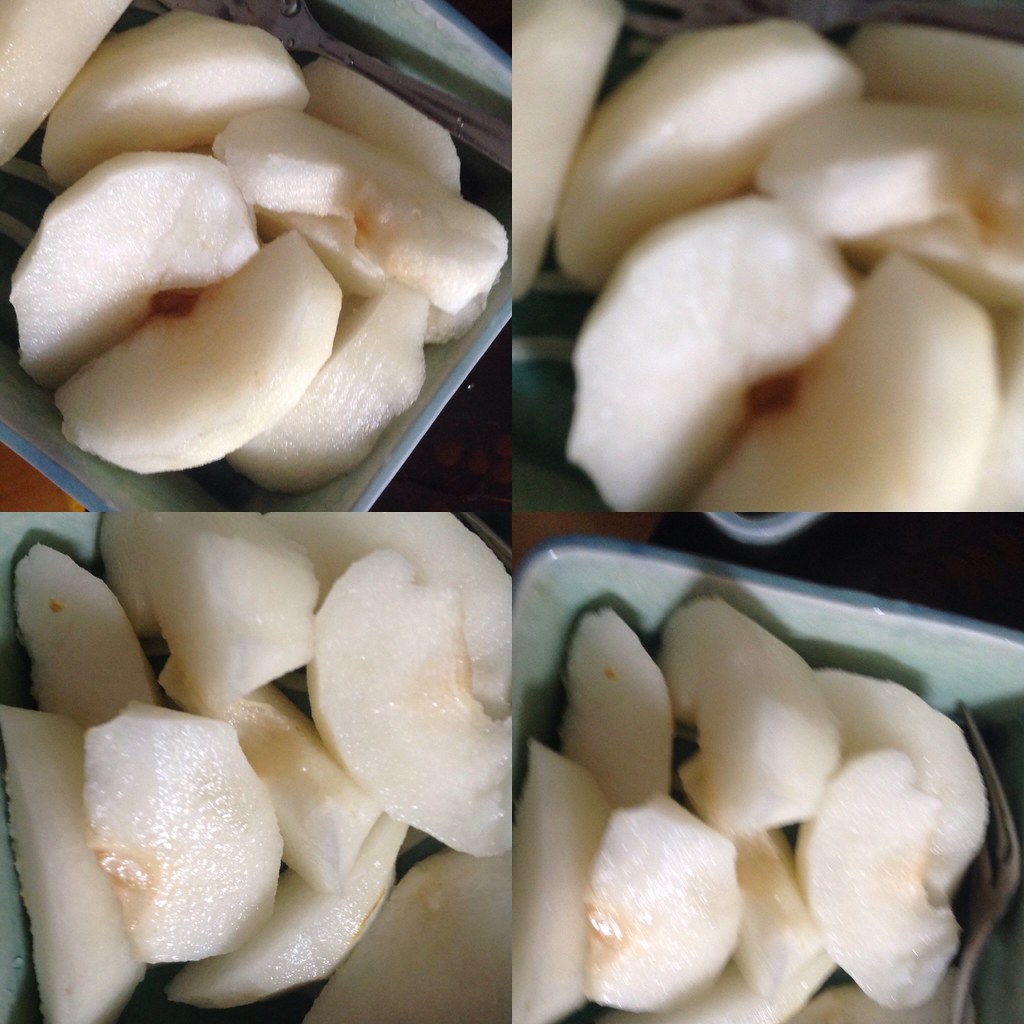This is a composite photograph divided into four panels, each displaying a close-up of sliced and peeled apples in a small, square, light gray ceramic dish. The apples have a white, moist texture and appear in a handful-sized pile in each image. The top left panel clearly shows the apples in the ceramic dish, and a fork is partially visible. The top right panel is a blurry close-up, obscuring details but still showing the apples and part of the dish. The bottom left panel provides a different angle of the apples in the same dish, while the bottom right panel features the apples with a tiny fork visible in the bottom right corner of the dish. All images are consistent in theme and setup, lacking any text, people, or animals.